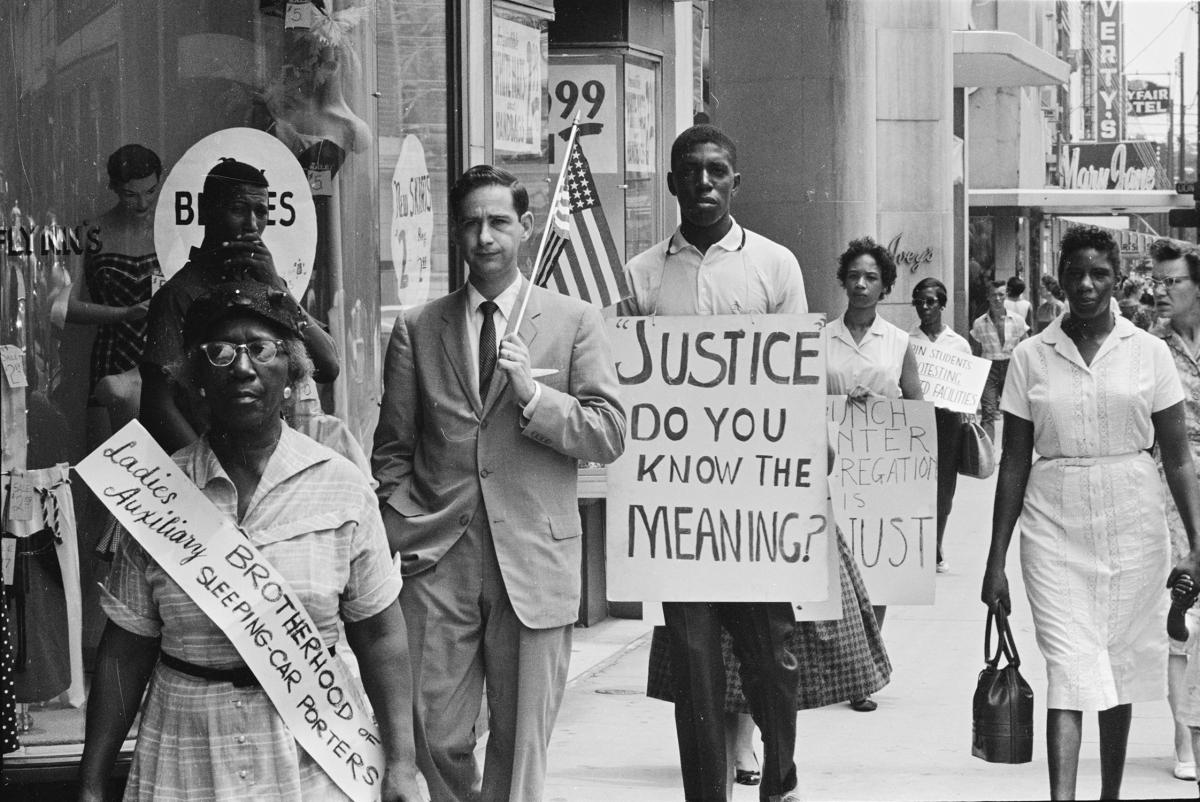In this detailed black-and-white photo from what appears to be the 1950s or 60s, a diverse group of civil rights protesters is marching down a busy city street lined with storefronts. Prominently in the foreground, an elderly black woman with glasses wears a shirt dress and a sash that reads "Ladies Auxiliary, Brotherhood of Sleeping Car Porters." Walking behind her is a Caucasian man dressed in a suit and tie, carrying an American flag in his left hand while his right hand rests in his pocket. Further back, a tall young black man in a collared sports shirt and slacks holds a white sign with bold black letters asking, "Justice, do you know the meaning?" Accompanying the group is a young black woman carrying a partially visible sign that mentions "Lunch Counter Integration." The crowded sidewalk features a mix of onlookers and other protesters, both black and white, some holding indistinguishable signs. The scene is rich with historical context, evidenced by the period attire and the emblematic messages advocating for civil rights.